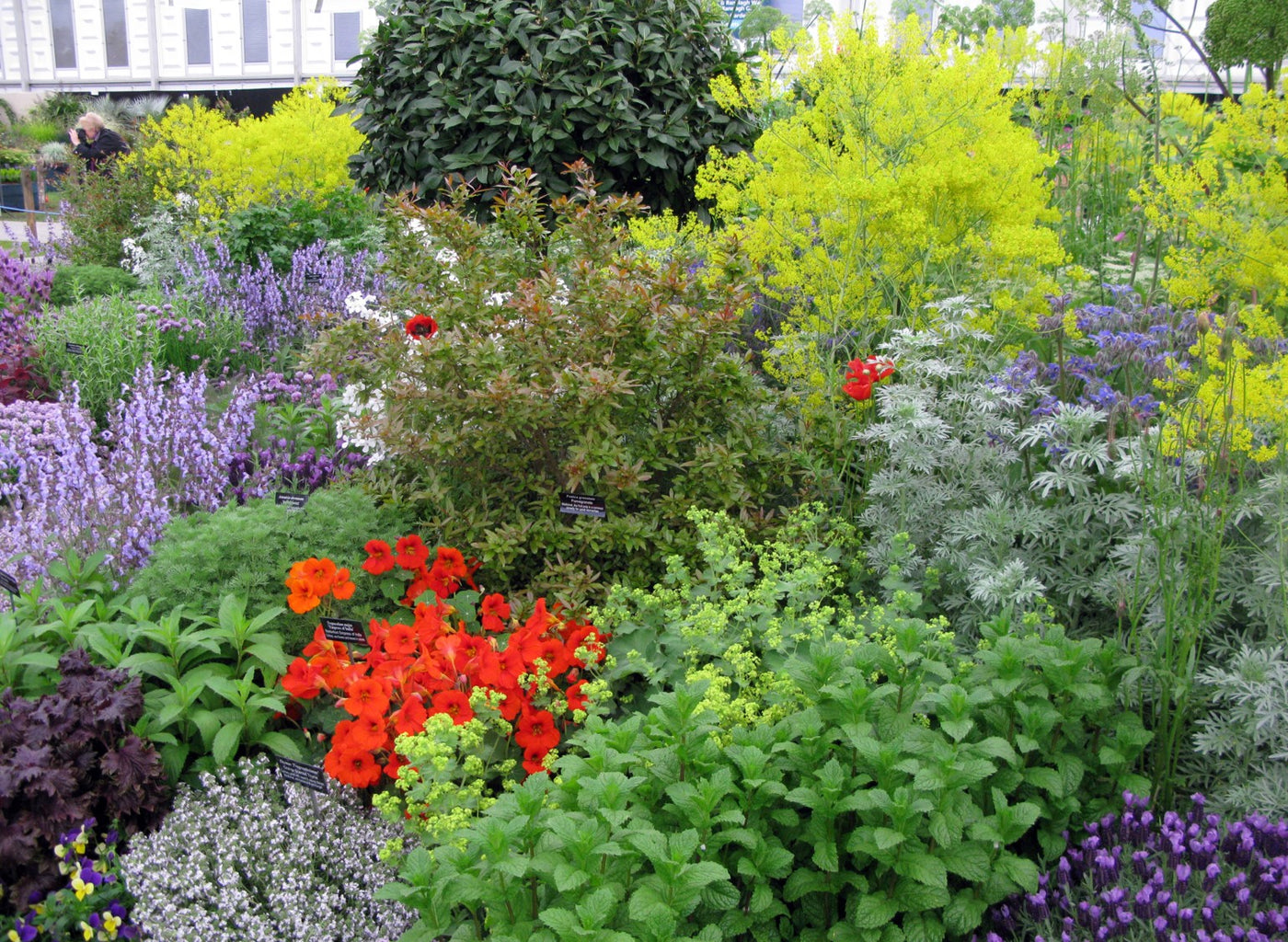The photograph captures a verdant garden brimming with various flowers and bushes, closely intertwined without any clear separation. Dominating the center of the top of the frame is a large green bush. To its right, there's a bush with yellowish-green leaves and, beneath it, a less lush greenish-brown bush boasting a single red and black flower. Scattered throughout the garden are vibrant clusters of flowers: bright red ones near the bottom left, numerous purple blooms mainly to the left and right, and pale yellow-green flowers near the bottom right, mingling with gray-leaved plants dotted with small purple flowers. Black tags with illegible white text are placed amongst many of the plants, indicating their types.

In the background, partially obscured by the lush garden, stands a large white building with rows of gray windows. Beneath the building, a woman with light blonde hair is slightly crouched forward, aiming her camera to the left of the frame. Her form is partially hidden behind a green bush, though it is clear she is intent on capturing the beauty surrounding her. In the top left of the image stands another woman, barely visible, with white hair and a black shirt, contributing to the scene with her presence.